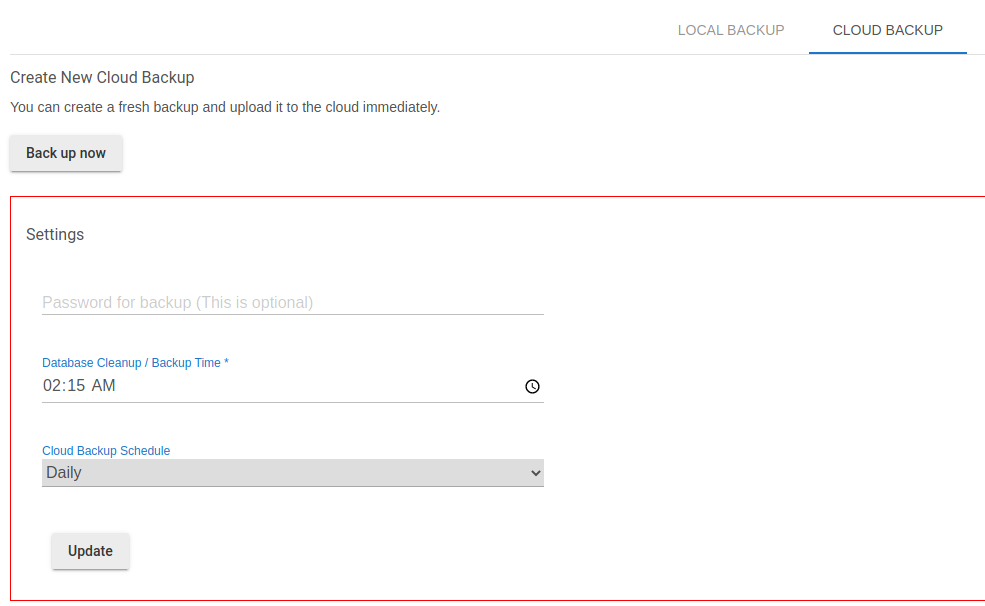This screenshot captures a segment of a website or software dashboard dedicated to backup management. At the top right, the interface features two distinct buttons labeled "Local Backup" and "Cloud Backup." Notably, the "Cloud Backup" text is highlighted with a blue underline, indicating it is currently selected.

Below this selection, a horizontal line separates this section from the next. On the left side of the line, the text "Create New Cloud Backup" is prominently displayed. Directly beneath this, there is an informative sentence that reads, "You can create a fresh backup and upload it to the cloud immediately." To facilitate this action, a gray button labeled "Backup Now" is situated below the descriptive text.

A red-bordered box highlights the area underneath these options, drawing attention to the settings section. The title "Settings" is positioned at the top left of this red box. Inside the box, there is an empty input field labeled "Password for Backup (optional)," suggesting that users can optionally secure their backup with a password.

Proceeding further down, labeled in blue text, "Database Cleanup / Backup Time" is displayed with a corresponding input field filled with the time "02:15 AM," indicating the scheduled time for this task. Below this, another blue label reads "Cloud Backup Schedule," accompanied by a dropdown menu set to "Daily," allowing users to specify the frequency of their cloud backups. At the bottom of this section, a gray "Update" button is available to save any changes made to the settings.